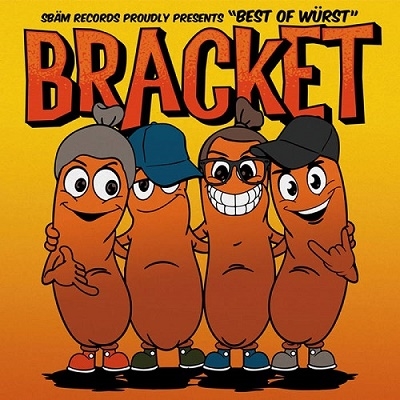This square cartoon image features four anthropomorphic sausages standing upright against a vibrant background that transitions from yellow at the top to orange at the bottom. At the top of the image, black text reads, "Spahn Records proudly presents," followed by, "Best of WÜRST," with "WÜRST" highlighted in quotations and spelled with a "U" featuring an umlaut. Below this, in large, capitalized orange letters with black shadowing, is the word, "BRACKET."

Each of the sausages is depicted with unique features and accessories, enhancing their individuality. From left to right:
1. The first sausage wears a gray hat and has big eyes, flashing a hang loose sign with its right hand. It is a brown sausage wearing red shoes.
2. The second sausage sports a blue baseball cap and green sneakers. It looks straight ahead with its mouth closed.
3. The third sausage smiles broadly, showcasing a toothy grin and nerd glasses. It has brownish-gray hair pulled back into a bun and wears blue shoes.
4. The fourth sausage wears a black baseball cap and is making a hand gesture, possibly a devil horn symbol, with its left hand. It has big eyes, an open mouth, and gray sneakers.

Beneath each sausage, there are black shadows that add depth to the cartoon. The overall aesthetic suggests this could be a cover for a book or comic book, bringing a playful and vibrant look to the characters and their setting.